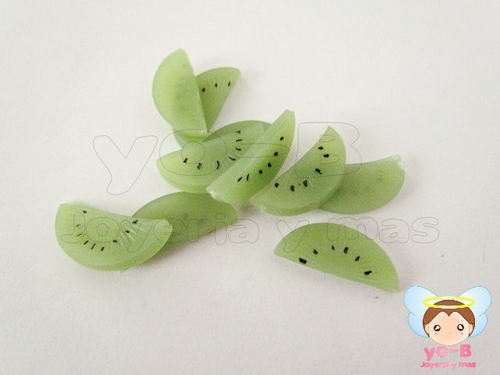This image features a small, square, pinkish-gray background with green kiwi slices scattered randomly across the center. Each kiwi slice is adorned with an arc of tiny black seeds. In the lower right corner, there's a cartoon figure of an angel with brown hair, a gold halo above her head, and bluish-white wings visible from behind. The angel, dressed in a pink outfit, has black and white dotted eyes. Below the figure is text that reads "Yo-B" and "Joyeria Emos" in pink letters. The kiwis, appearing to be slices from one whole fruit, are laid out haphazardly, with some overlapping and others spread out separately.